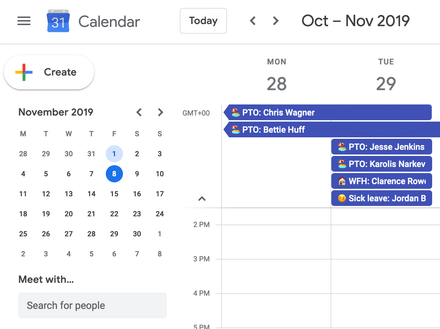The image displays a Google Calendar interface with a detailed header and split content. The header features three small horizontal lines on the far left, indicating a drop-down menu. Adjacent to this is a blue icon resembling a flip desk calendar with the number '31' in gray. Beside the icon is the word "Calendar." Centrally located within the header is a button labeled "Today" in black with a rectangular outline, flanked by left and right arrowheads for navigation. Continuing to the right, the header shows the abbreviated months "OCT" and "NOV" for October and November 2019, respectively.

Beneath the header, the page is divided into two sections. The left section features a "Create" button with the Google plus sign. Below this button is a mini-calendar for November 2019, highlighting Friday, November 1st with a light blue circle and Friday, November 8th with a dark blue circle. All other dates are displayed in black without circles. Underneath the mini-calendar, the text "Meet with" appears, followed by a light gray search box for finding people.

The right section presents a detailed day-by-day view. At the top, the abbreviations for Monday ("MON") and Tuesday ("TUE") are displayed with the dates "28" and "29" underneath them, respectively. The calendar illustrates the schedule from midnight to 5 p.m. It includes two all-day PTO requests for both Monday and Tuesday. Additionally, Tuesday's schedule lists two more PTO requests, a work-from-home request, and a sick leave request. There are no entries in the time slots from 2 p.m. to 5 p.m.